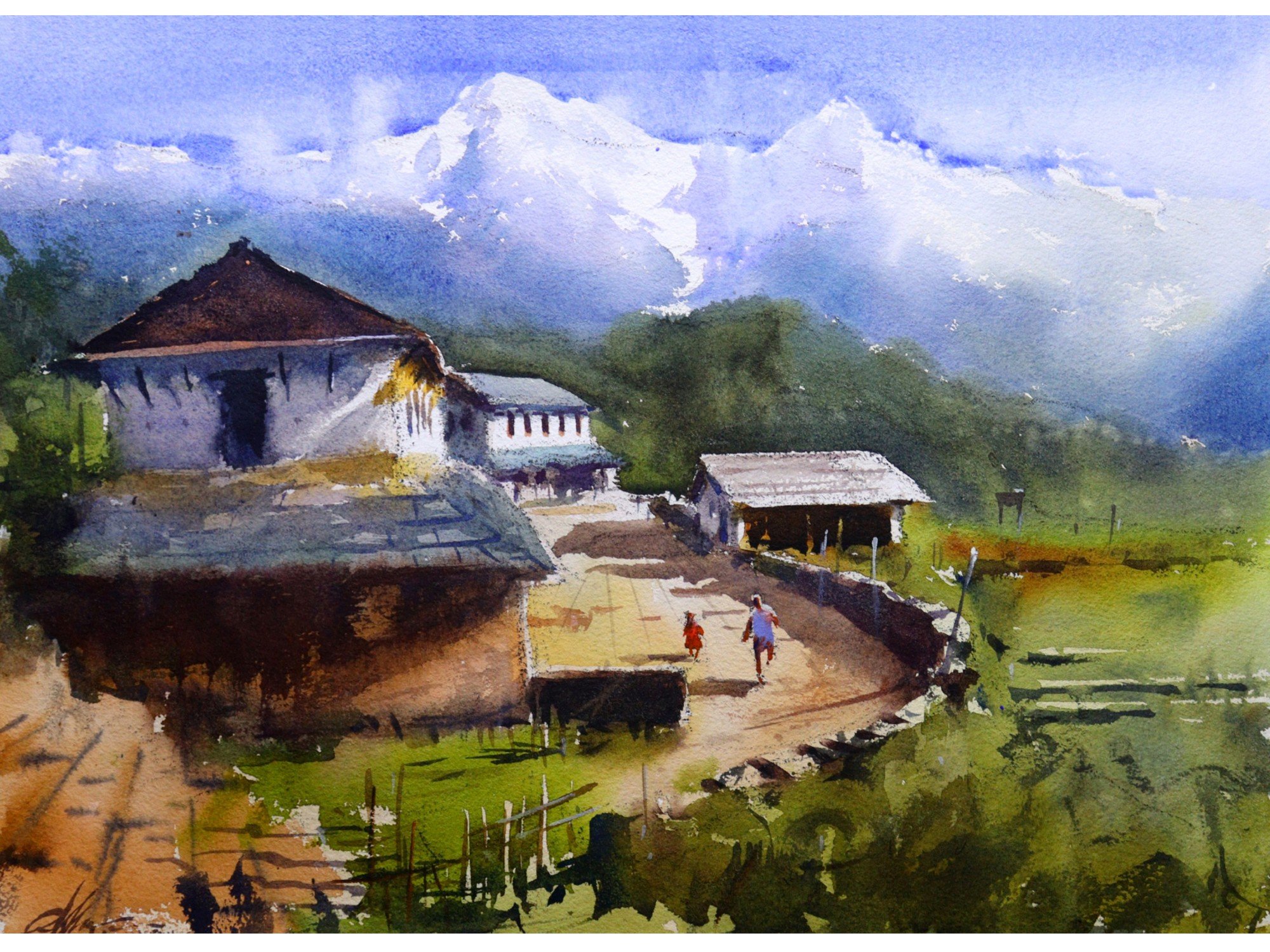This painting features an abstract and colorful depiction of a farm-like landscape. In the background, snow-capped white mountains rise majestically against a blue sky, adorned with wisps of white clouds. Below the mountains, a belt of tall green trees reaches up to mid-mountain height. 

Foreground elements of the painting showcase several buildings: a prominent large white house with black windows and a blue awning, and another with a tall, brown, triangular roof and an open window. There is also a white and tan cabin reminiscent of a barn. The painting includes a light yellow or tan stone pathway winding through the scene, on which an adult dressed in blue and a child in red are running or walking.

To the right of the charted pathway, a sprawling, colorful green field is divided by a middle fence, while a small shed is visible nearby. The fields exhibit various shades of green and brown, with black shadows adding depth and texture. Despite the sloppy and imprecise brushstrokes typical of watercolor, the painting brims with vivid colors and an impressionistic style, capturing the serene yet dynamic beauty of this rural landscape.